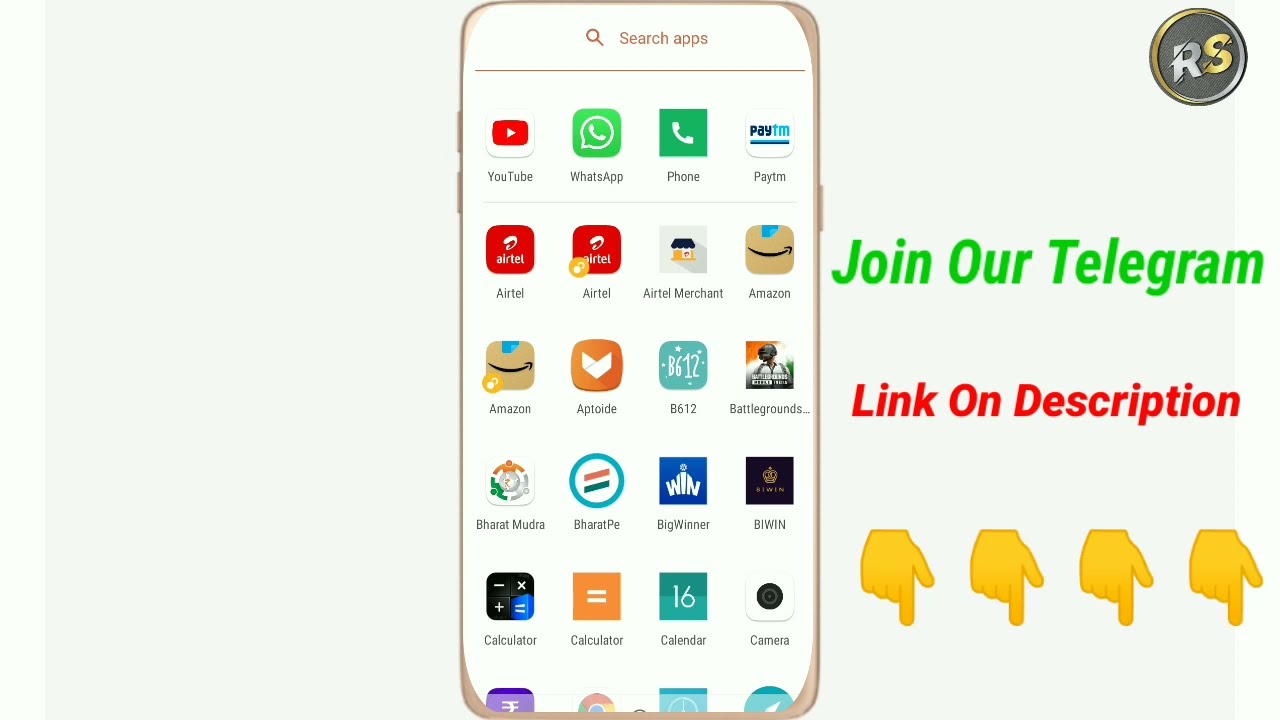This image portrays a detailed, computer-drawn representation of a cell phone screen set against a white background. At the top of the screen, the text "search apps" is displayed, followed by a series of app icons that include YouTube, WhatsApp, Phone, Paytm, Airtel, Airtel Merchant, and Amazon, among others. Additionally, there are icons for Calculator, Calendar, and Camera, though some icons are unclear. 

In the upper right corner of the screen, there is a circular logo with the initials "RS" — the "R" is silver and the "S" is gold. Below this logo, on the right side of the image, "join our telegram" is prominently written in green text, followed by "link on description" in red text. Below this text, four yellow hands are pointing downwards, directing viewers to the described link.